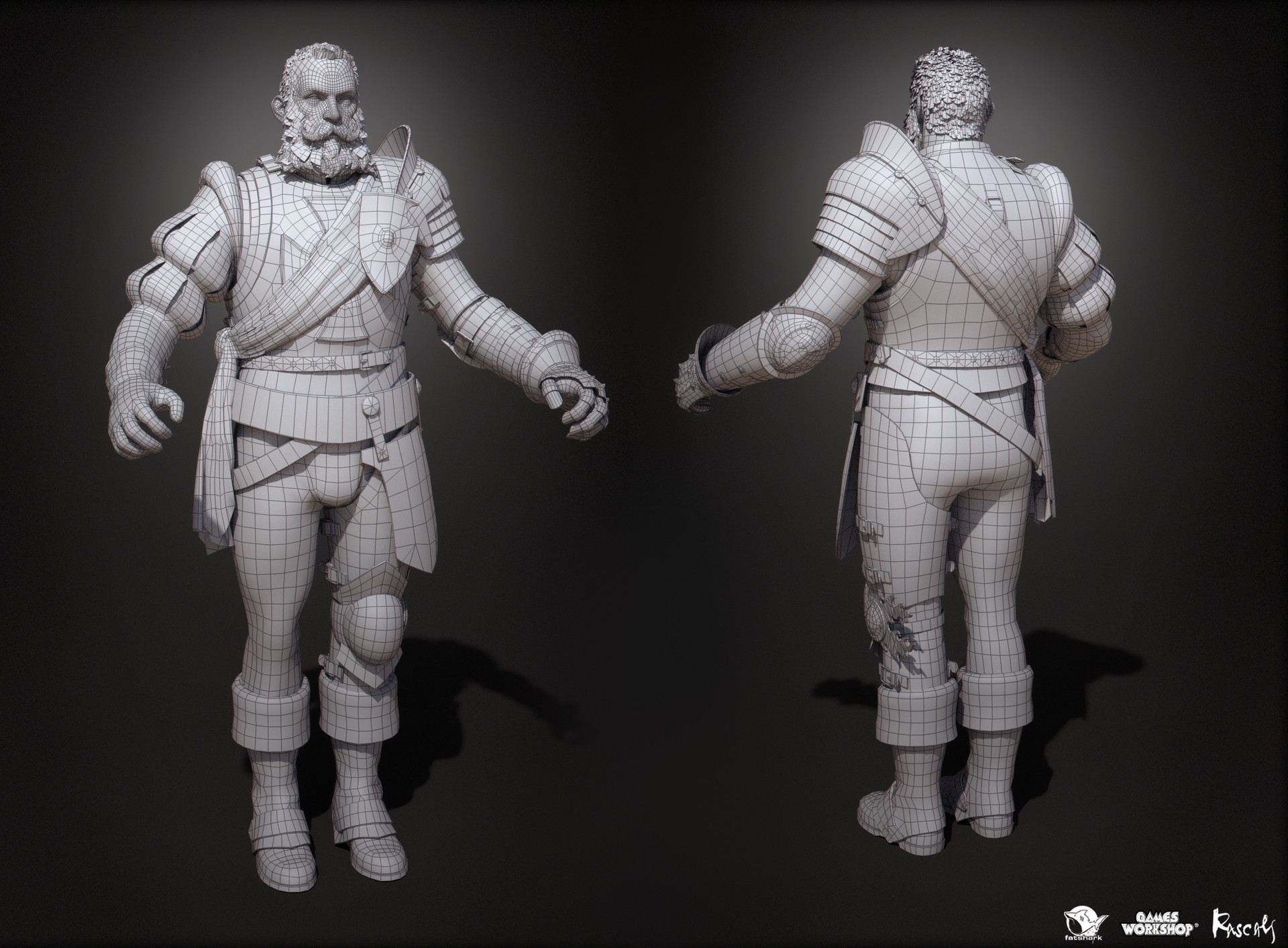The image in question is a computer-generated black and white square illustration with no borders. The background is predominantly black, transitioning to a lighter shade towards the center, giving a gradual gradient effect. In the lower left corner, there's a white text that reads "Games Workshop" along with an undecipherable round logo and a handwritten signature that appears to say "R-A-S-C-H-K-Y."

The main focus of the image is a character model rendered in a 3D software, likely intended for movies or video games. The character, who looks like an elderly man with a thick, formal-looking beard and short curly hair, is dressed in old-fashioned attire featuring a sash across his chest, poofy sleeves, and an armor-like garment. The image showcases front and back views: the left side displays the front, and the right side displays the back. The character’s arms are extended sideways with palms facing down, and the entire body is covered with a light gray grid pattern, indicating the model's wireframe structure.